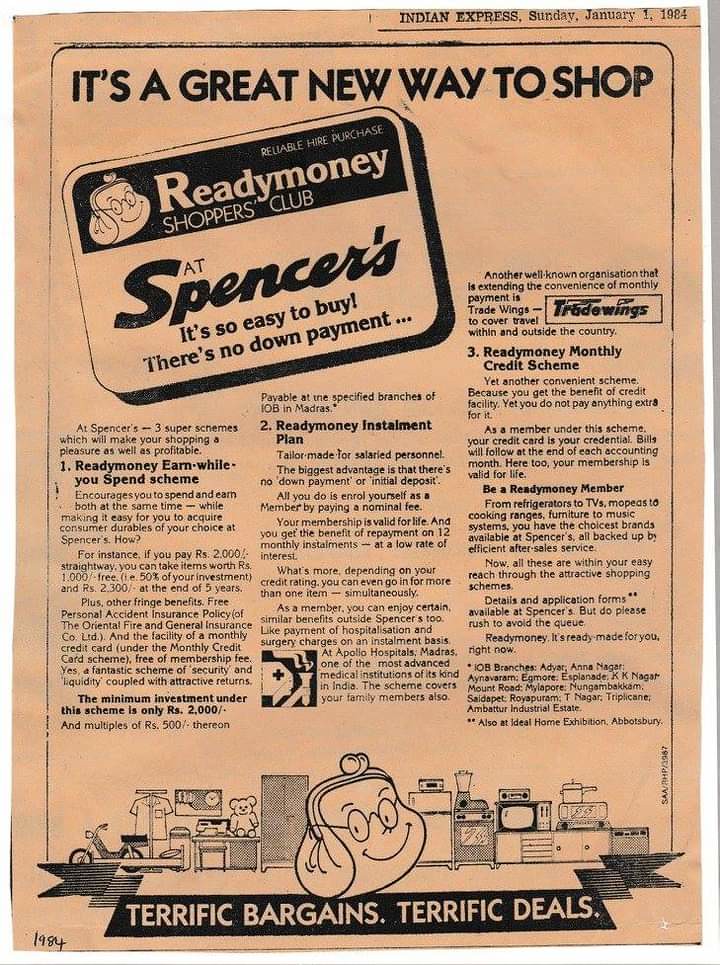This is a detailed depiction of a full-page advertisement from the 'Indian Express' dated Sunday, January 1st, 1984. The ad is printed on a tan-colored paper with black text and illustrations. At the top, it proclaims "It's a great new way to shop" and just below, prominently features "Ready Money Shoppers Club at Spencer's" within a rectangle with rounded edges. The tagline "It's so easy to buy, there's no down payment" underscores the ease of purchasing.

The ad categorizes its offers under three main schemes detailed in three columns of fine print:
1. **Ready Money Earn While You Spend Scheme**: Encourages earning while spending. For example, paying RS-2000 upfront allows you to take items worth RS-1000, obtaining substantial returns coupled with added benefits such as free accident insurance.
2. **Ready Money Installment Plan**: Designed for salaried personnel, eliminating down payments or initial deposits, and offers the flexibility of repaying in 12 monthly installments at low interest rates. The scheme provides life-long membership and benefits including medical expenses coverage at Apollo Hospitals.
3. **Ready Money Monthly Credit Scheme**: This scheme offers the convenience of monthly credit without extra costs. Membership is valid for life, enabling purchasing from a range of products from refrigerators to furniture with substantial after-sales services.

At the bottom, an illustration depicts a smiling face surrounded by various consumer goods such as a television, blender, teddy bear, refrigerator, clothes, and bicycles, showcasing the vast array of available products. The advertisement wraps up with a call to action, encouraging potential customers to take advantage of "terrific bargains, terrific deals." The additional details include the locations where the scheme can be availed across various IOB branches in Madras. 

Overall, this vintage ad encapsulates an attractive, no-hassle shopping experience at Spencer's with multiple beneficial schemes aimed at consumer convenience.